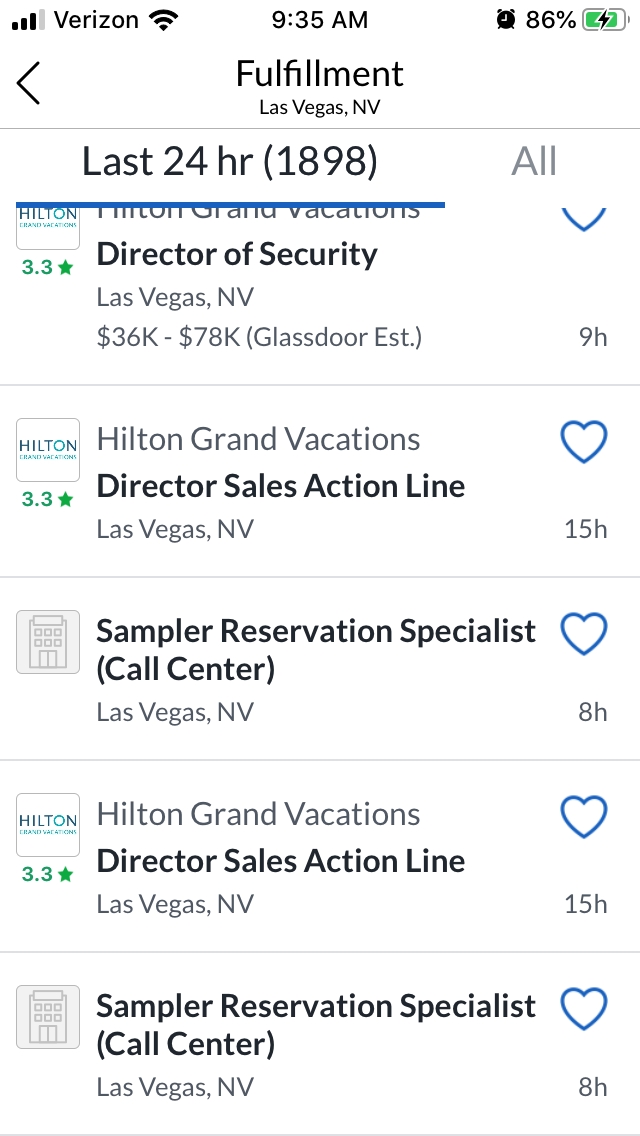This is a screenshot featuring a job listings app interface specifically for recently posted job opportunities. The background is a clean white, and at the top center, the heading reads "Fulfillment, Las Vegas, Nevada." To the left of this heading, there's a back arrow icon. Below this, a subheading displays "Last 24 Hours," with a count of "1898" listings. On the right side of the subheading is an "All" dropdown box for filtering options.

The main section of the screen presents job listings in a vertical format. The first listing is for "Hilton Grand Vacations" advertising a "Director of Security" position in Las Vegas, Nevada, offering a salary range of $36,000 to $78,000 according to a Glassdoor estimate. This listing was posted 9 hours ago. In the top right corner of this listing, there is a heart icon allowing users to save the job post for later.

The second listing is also from "Hilton Grand Vacations" for a "Director of Sales, Action Line" role in Las Vegas, Nevada. This listing has a similar heart icon for saving the job and was posted 15 hours ago. To the left of these posts, there is a small thumbnail image representing the company along with a rating of 3.3 stars given by employees on the app.